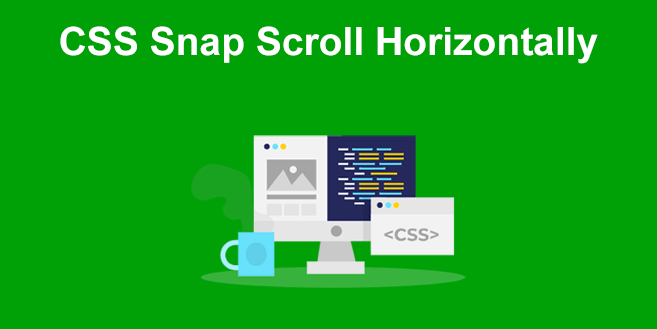A bright lime-green rectangle serves as the background, slightly muted in intensity. In the upper region, bold white text in a font size of approximately 24 points reads, "CSS Snap Scroll Horizontally." Centered towards the bottom of the rectangle is a digitally rendered image of a computer screen, split into two sections.

The left section of the screen displays stylized text represented by various colored lines: white, turquoise, and orange. The right section features a white background with three circles at the top in black, blue, and yellow, followed by the Instagram-like icon of a mountain.

The base of the screen rests in a semi-transparent shaded oval, giving it a subtle 3D effect. Nearby, a light turquoise coffee cup sits, marked by a simple circular pattern.

Additionally, there's an inset pop-up image of a white box with light gray shading around the edges. This box includes the same three colored circles at the top and two arrows facing each other inside. The letters "CSS" are prominently displayed within this pop-up box, signifying thematic consistency with the main caption.